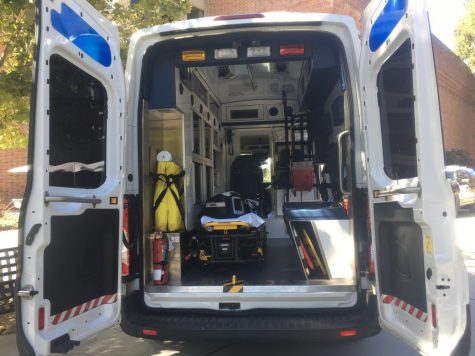The photograph captures an outdoor scene featuring an overcast sky with white clouds serving as a backdrop to a washed-out red brick building and the top portion of a tree on the left side. The main focus of the image is the back of an ambulance, which stands taller than it is wide, with both its doors open, revealing the interior. The ambulance doors have a blue tinted section at the top and dark, blacked-out windows. The bottom of the doors is marked with red and white stripes. Inside, a fire extinguisher is positioned at the lower left near the doorway, and a stretcher extends out like a shelf on the right. Affixed to the rightward wall is a tufted seat, and above it hangs a reflective yellow garment. The top interior section of the ambulance features four emergency lights: an orange one on the left, two white ones in the middle, and a red one on the right. The photograph also gives a glimpse of the driver's seat far in the distance, as well as some medical machinery and overhead lighting.